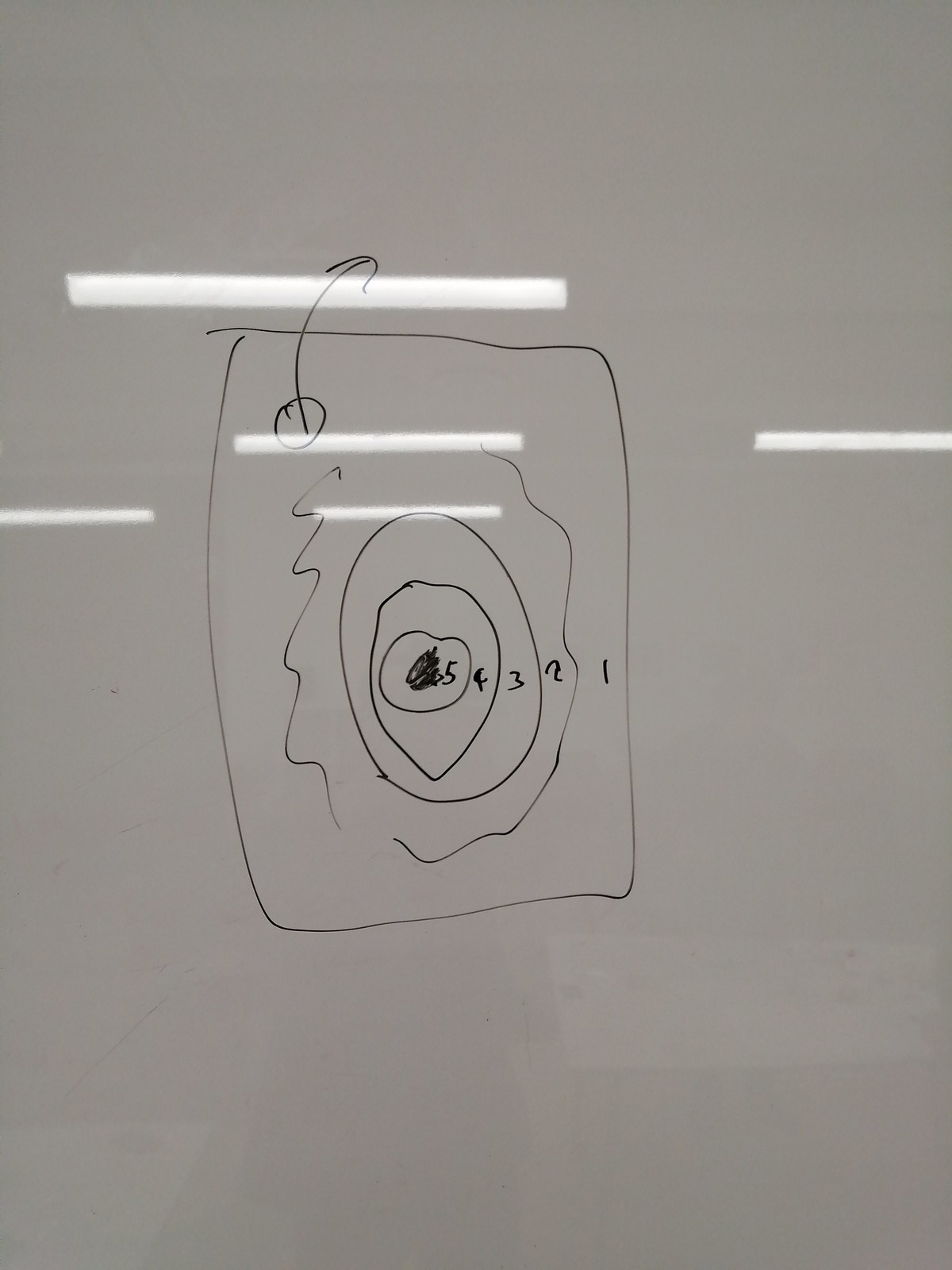Here we see an intricately detailed drawing on a white piece of paper, which also bears a few faint black marks in the bottom left corner. Another object seems to be faintly visible from the other side of the paper, subtly bleeding through. 

The central focus of the drawing is a large box shape located in the center of the page. This box has a hole at its top left corner, from which a black arrow emerges, pointing towards the top of the page. The entire drawing is rendered in what appears to be black ink or marker.

Inside the box, there are multiple wavy lines and a series of concentric circles, along with three distinct circles neatly positioned. The circles are encircled by wavy lines on both the left and right sides. At the very center of the design is a black circle marked with the number "5." Surrounding it, in order, are circles labeled "4," then "3," and "2" as one moves outward. Finally, on the outermost level on the right-hand side of the page, the number "1" is displayed.